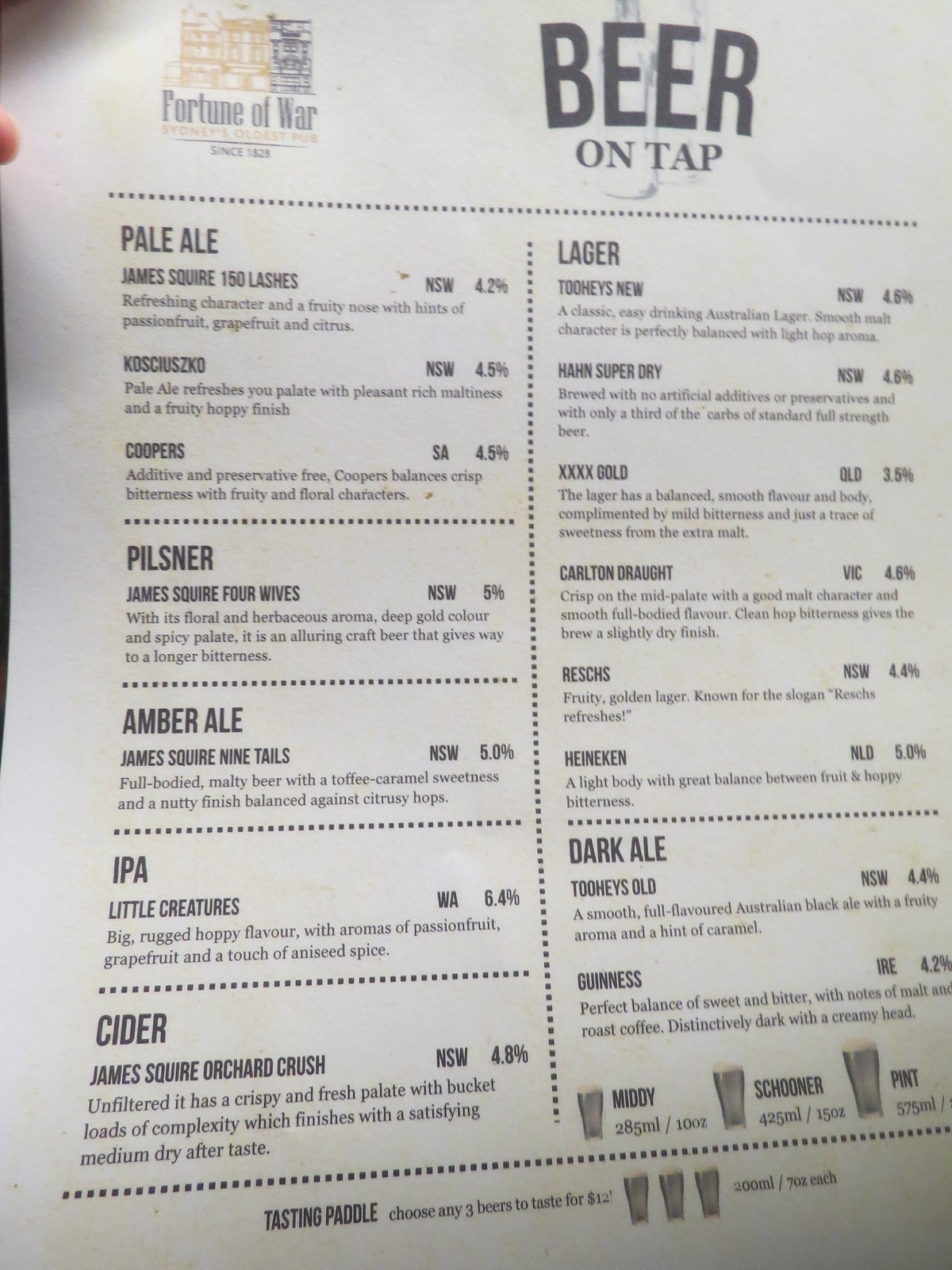The image is a color photograph in portrait orientation, showcasing a detailed beer menu from a place called Fortune of War, reputedly Sydney's oldest pub since 1828. At the top left, there is a beige and gray logo illustrating several buildings along with the establishment's name. Adjacent to this logo is a light gray icon of a beer mug, beside the large, bold, capitalized words "Beer on Tap." 

Below the heading, a horizontal line of dots is followed by a vertical line of dots, splitting the menu into two columns. The left column starts with "Pale Ale" and lists three beers, followed by single entries for "Pilsner," "Amber Ale," "IPA," and "Cider." The right column lists six "Lagers" and then two "Dark Ales," each beer accompanied by descriptions, origin details, price, and alcohol content. 

At the bottom of the menu, there is a size chart illustrating three different beer glass sizes: Middy, Schooner, and Pint. Additionally, there is a tasting panel offer suggesting a selection of any three beers for $12, with specific ounce information for each tasting glass. The overall style of the menu is photographic representationalism realism.